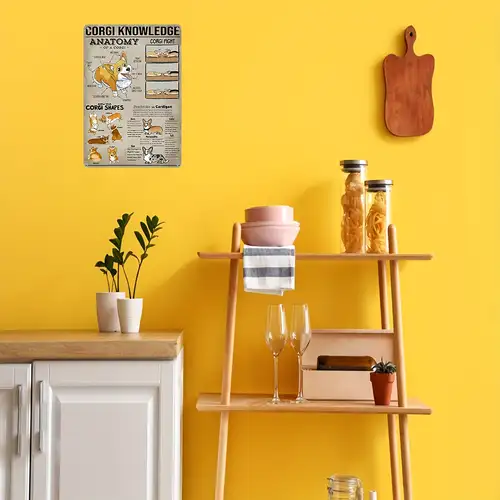This photograph captures a cozy corner of a room with a mustard-colored wall adorned with various decor items. On the upper left of the wall is a poster titled "Corgi Knowledge," featuring a detailed cartoon-style drawing of a corgi dog, along with smaller illustrations and anatomical details about corgis. To the right of the poster, a wooden cutting board shaped somewhat like a guitar body hangs on the wall.

Below these wall hangings is a white cabinet with a natural wood grain countertop. Atop the cabinet are two small white vases, each containing a sprig of green leaves. To the right of the cabinet is a set of shelves. The top shelf showcases glass jars filled with dried pasta, some bowls, and a white-and-gray striped dish towel. The lower shelf holds two wine glasses, a small terracotta pot with a plant, and a box that appears to contain a bottle of wine. The arrangement of these items creates a rustic and homely atmosphere in this section of the room.